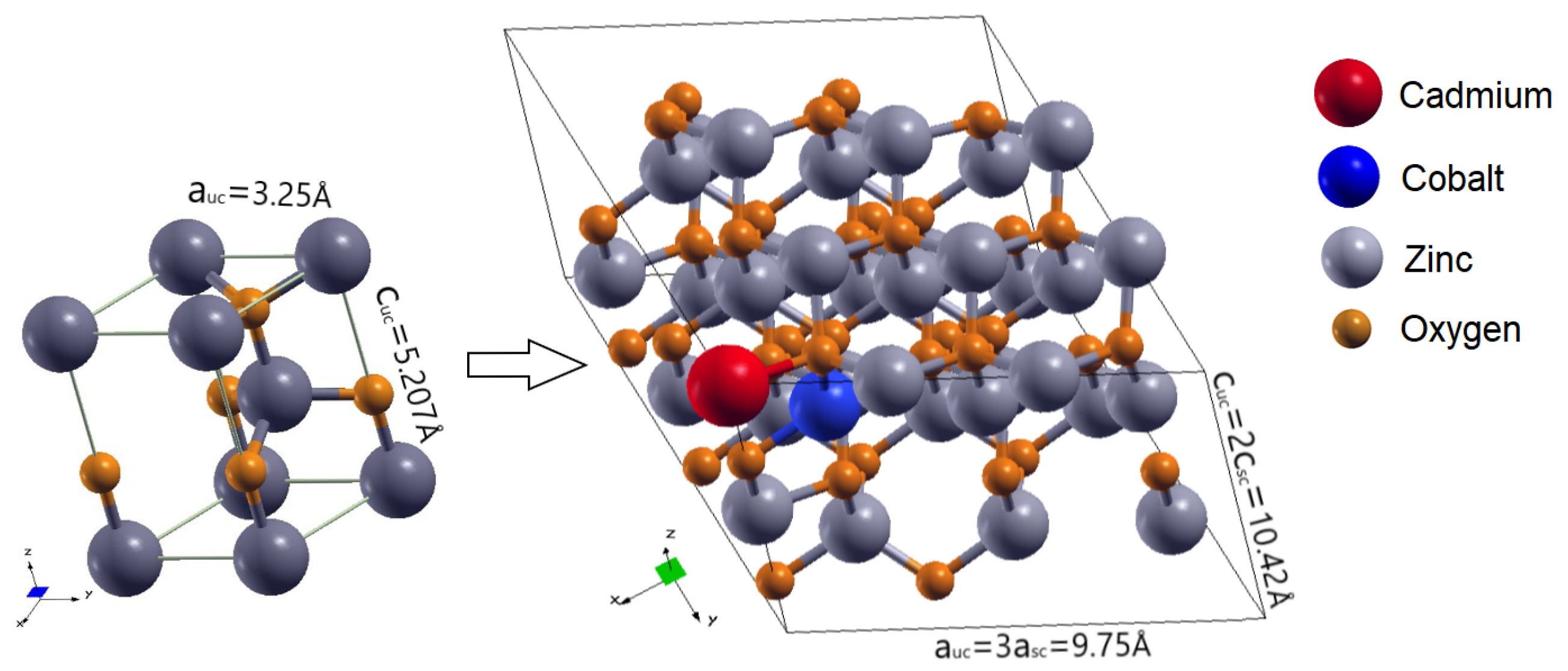The image depicts a scientific diagram featuring molecular structures with diverse colored spheres. On the left, a cube structure is formed by gray zinc atoms at its vertices, each joined by smaller golden oxygen atoms. This cube is annotated with formulas such as "AUC = 3.25" and "CUC = 5.207A." An arrow points from this cube to a larger, more complex structure in the center, which contains a mix of periwinkle zinc atoms, and is interspersed with smaller golden oxygen atoms, a red cadmium atom, and a blue cobalt atom, arranged in a seemingly random pattern. Equations such as "AUC = 3" and "SC = 9.75A" accompany these structures. To the bottom left of the central cluster, a legend indicates the element each color represents: red for cadmium, blue for cobalt, gray for zinc, and gold for oxygen. The intricate connectivity and annotations highlight this as a detailed scientific representation.